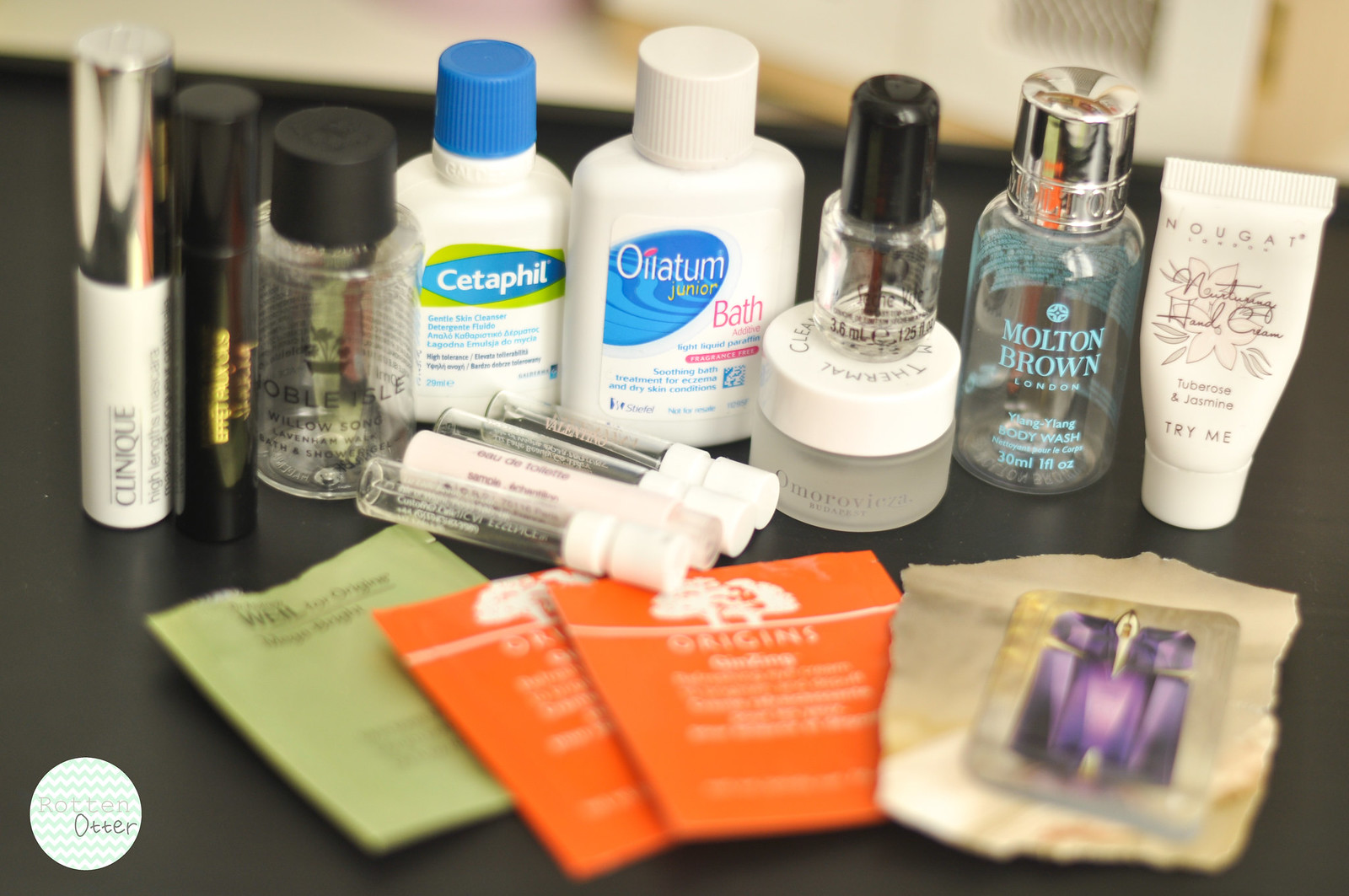The photograph displays an assortment of beauty products meticulously arranged on a dark gray counter against an ivory background. It appears either as a personal collection or a store display, featuring a variety of brands and items. Positioned at the lower left corner is a circular label with the word "OTTER."

Starting from the left, there is an upright tube labeled "Clinique." Next to it stands a sleek black tube. Adjacent to these is a clear bottle, seemingly marked "Noble Isle," topped with a black lid. Moving right, there is a solid white plastic bottle branded "Cetaphil," distinguished by its blue cap.

Following that, a white plastic bottle with a white cap bears the label "OILA TUM Junior Bath." Beside it, a circular container with a white top supports a smaller, clear jar capped in black. Further right, a clear jar marked "Molton Brown London" sports a silver cap, standing next to a white hand cream labeled "NOUGAT."

Lying horizontally beneath this collection are four small, lidded vials. In the foreground, three envelopes are positioned flat on the counter; one is tan with a torn top, and the other two are orange with white writing. Completing the scene is an ivory piece of paper featuring some purple detailing.